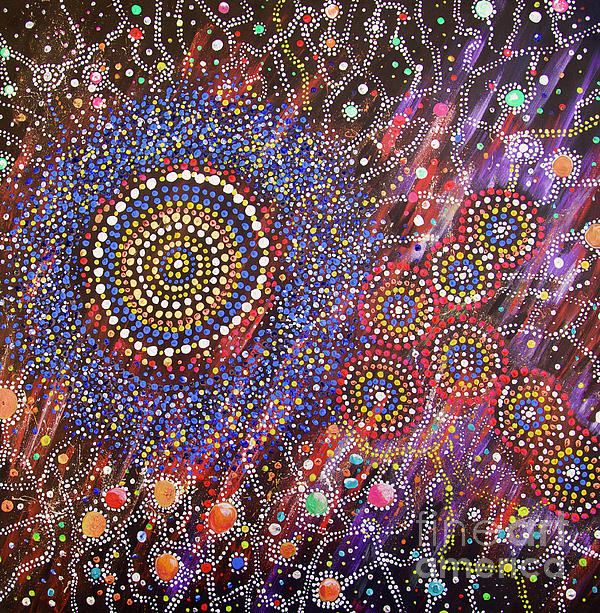The image is a vibrant and highly colorful representation, resembling a beaded artwork but potentially a painting. Dominating the scene is a large starburst pattern on the left side, bursting with yellow, blue, red, and white hues reminiscent of fireworks. This central figure radiates with smaller concentric circles featuring a mix of blue and yellow.

Surrounding the starburst are numerous smaller circles with white centers, interspersed with varying colors such as blue, yellow, pink, white, and red. These smaller elements trail off from the central explosion, creating a sense of dynamic motion.

The background is filled with streaks of vivid colors and an array of plain circles in pink, green, orange, yellow, and red, adding to the chaotic yet harmonious blend of the composition. Fine Art America's watermark is located in the bottom right corner, indicating the source or copyright of this captivating piece.